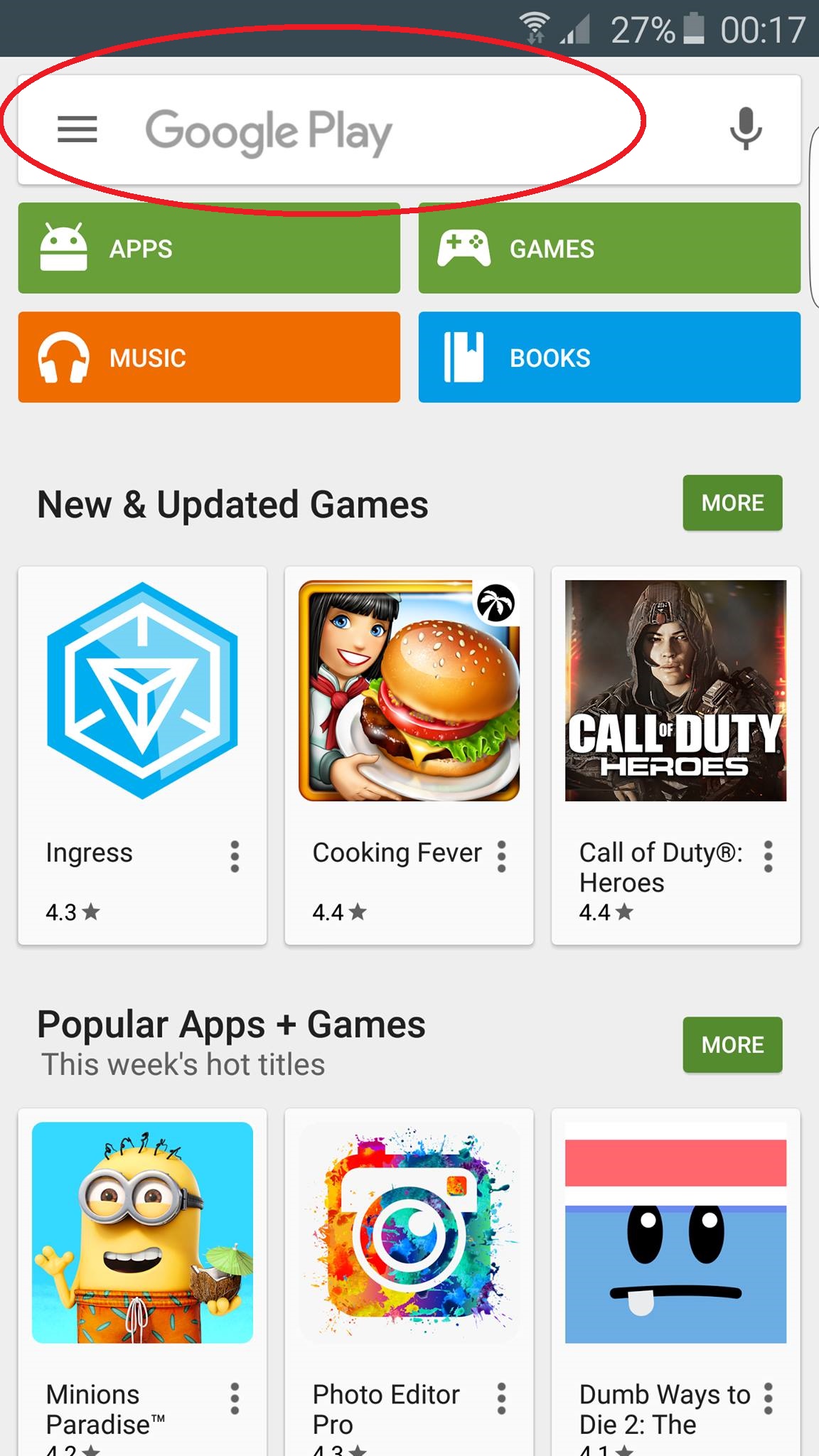This screenshot of a mobile phone displays the Google Play Store interface. At the very top, a gray status bar provides information about the device: the Wi-Fi signal is full, but the mobile signal shows only two out of four bars, the battery is at 27%, and the time reads 00:17. Directly below the status bar, the header of the Google Play Store is visible within a white rectangle outlined in gray, with the text "Google Play" circled in red. To the right of this text is a microphone icon for voice search functionality.

Beneath the header are four color-coded rectangles representing different sections: two green ones on the top row and a red and blue one on the bottom. The upper left green rectangle, labeled "Apps", features a white alien icon. To its right, the green rectangle labeled "Games" displays a white game controller icon. Below "Apps", the red rectangle labeled "Music" includes a white headphones icon. To the right of "Music," the blue rectangle labeled "Books" is marked with a white book icon. Following these sections, the text "New and updated games" appears in black font, indicating the latest offerings available in the Play Store.